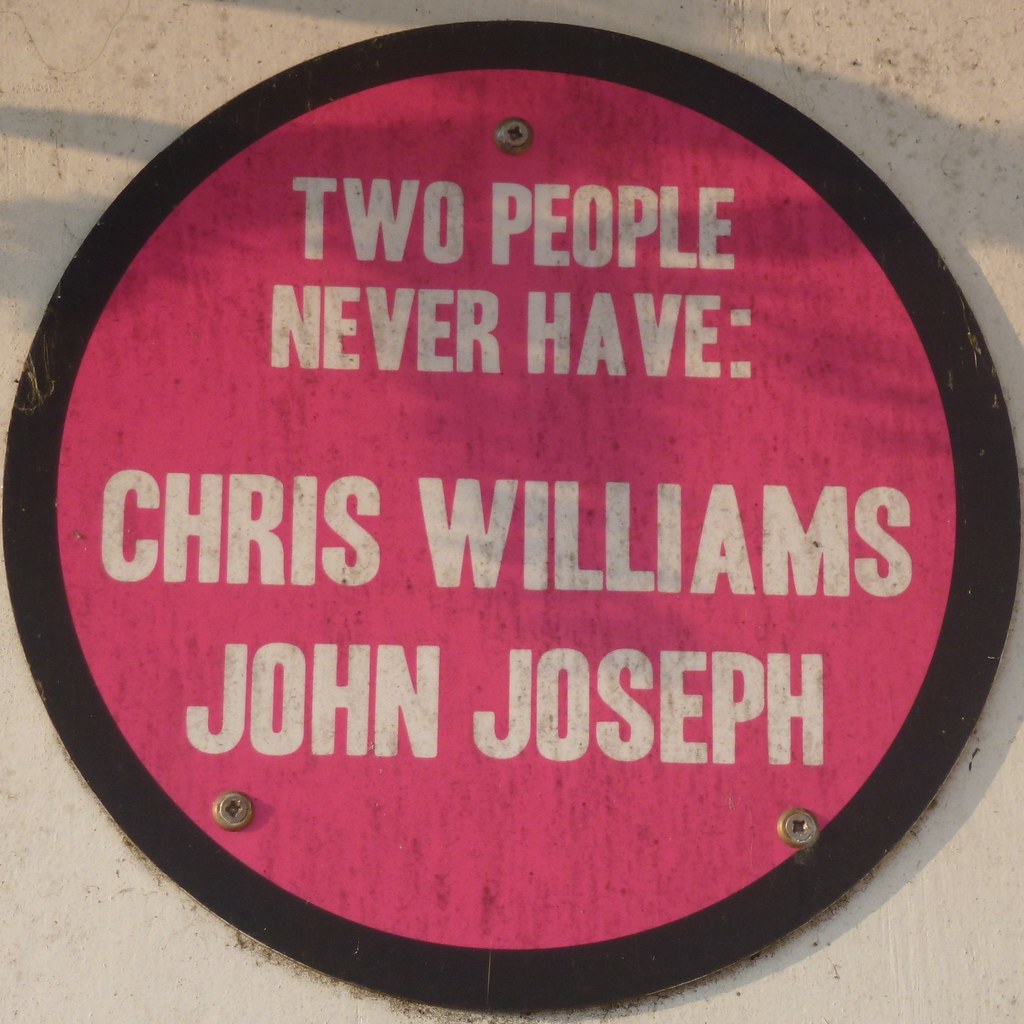The photograph captures a striking outdoor scene, featuring a circular sign prominently bolted to a light cream or off-white wall, which appears slightly pitted yet well-maintained. The wall textures look somewhat like stone or concrete. Shadows play across the image, adding depth and contrast. The circular sign itself, which occupies most of the frame, has a vivid design: a black border encircles its bright pink interior. White capital letters on the sign read, "TWO PEOPLE NEVER HAVE:", followed by the names "CHRIS WILLIAMS" and "JOHN JOSEPH" arranged vertically. Three Phillips head screws are visible, securing the sign: one positioned at the top center and two at the bottom near the names, specifically below the "J" in "John" and the "H" in "Joseph". There appears to be some dirt or dust collected around the lower rim of the sign, enhancing the sense that it's been there for some time.